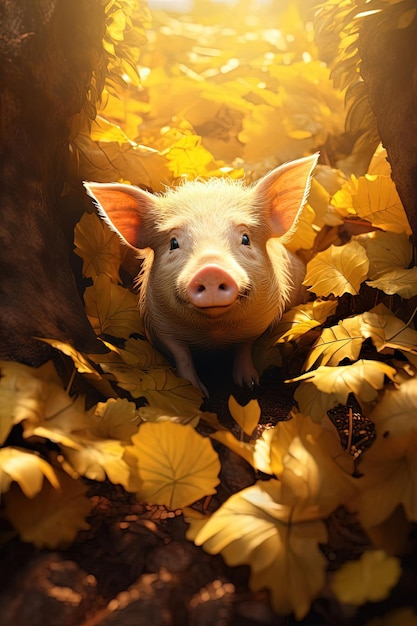A highly detailed and photorealistic image depicts an adorable pig, which appears to be computer or AI-generated. The pig, with its cute little black eyes, gazes directly at the viewer. Immersed in a bed of autumn leaves, the pig seems to be enjoying itself, surrounded by a sea of vibrant yellows. Sunlight streams in from above, casting a warm glow over the scene and highlighting the leaves in a visually pleasing manner. The image radiates strong autumn vibes, capturing the essence of the season. The pig appears to be having a wonderful time, frolicking through the forest leaves, and its joyful expression suggests it is delighted to encounter the viewer at this moment.